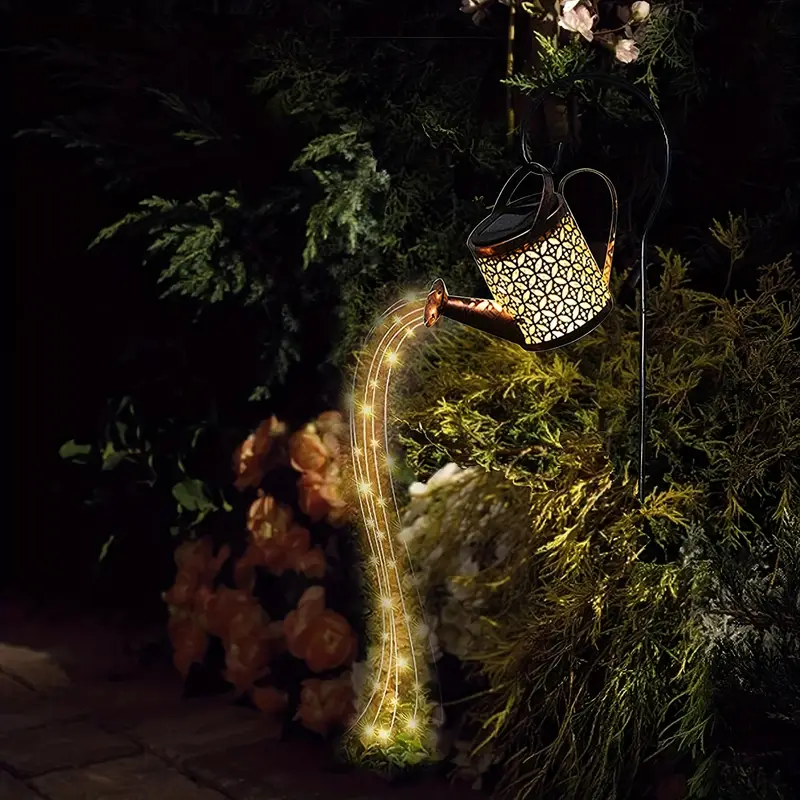This nighttime photograph, set in a garden area, showcases a unique decorative feature in a dimly lit atmosphere. On the right side, a black metallic pole stands erect, curving gracefully at the top to support a whimsical watering can lantern. The watering can, cream-colored with black accents, emits a cascade of golden light resembling water, which pours down, illuminating the ground below with sparkling yellow stars. Surrounding this enchanting focal point are lush green and light green plants, adorned with striking orange-yellow flowers. The pathway, visible at the bottom left corner, is brown and contrasts with the greenery and decorative structure. The scene blends a mix of real and possibly CGI elements, creating a magical ambiance that enhances the garden's visual appeal.